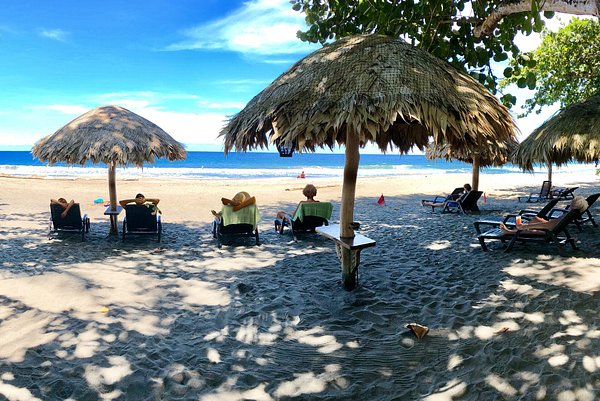This picturesque photograph captures a serene tropical beach scene on a bright, sunny day with a few scattered clouds dotting the vivid blue sky. The viewer appears to be standing in the shade, perhaps beneath a large tree with numerous leaves that frame the top of the image. In front, the sandy expanse is marked by countless footprints that lead to a wide and long beach, ending at a sharply blue ocean. Several straw umbrella-like structures, likely crafted from real or fake palm fronds and supported by thick wooden poles, provide shade to small tables beneath them. Under these umbrellas sit at least six lounge chairs, occupied by people lounging comfortably with their backs to the viewer, gazing at the tranquil sea. Some of the people have drinks, enhancing the relaxed and leisurely vibe. The vibrant colors of the beach and ocean, combined with the chairs aligned neatly under the shaded huts, evoke a deeply peaceful and inviting atmosphere, making it a perfect tropical escape.